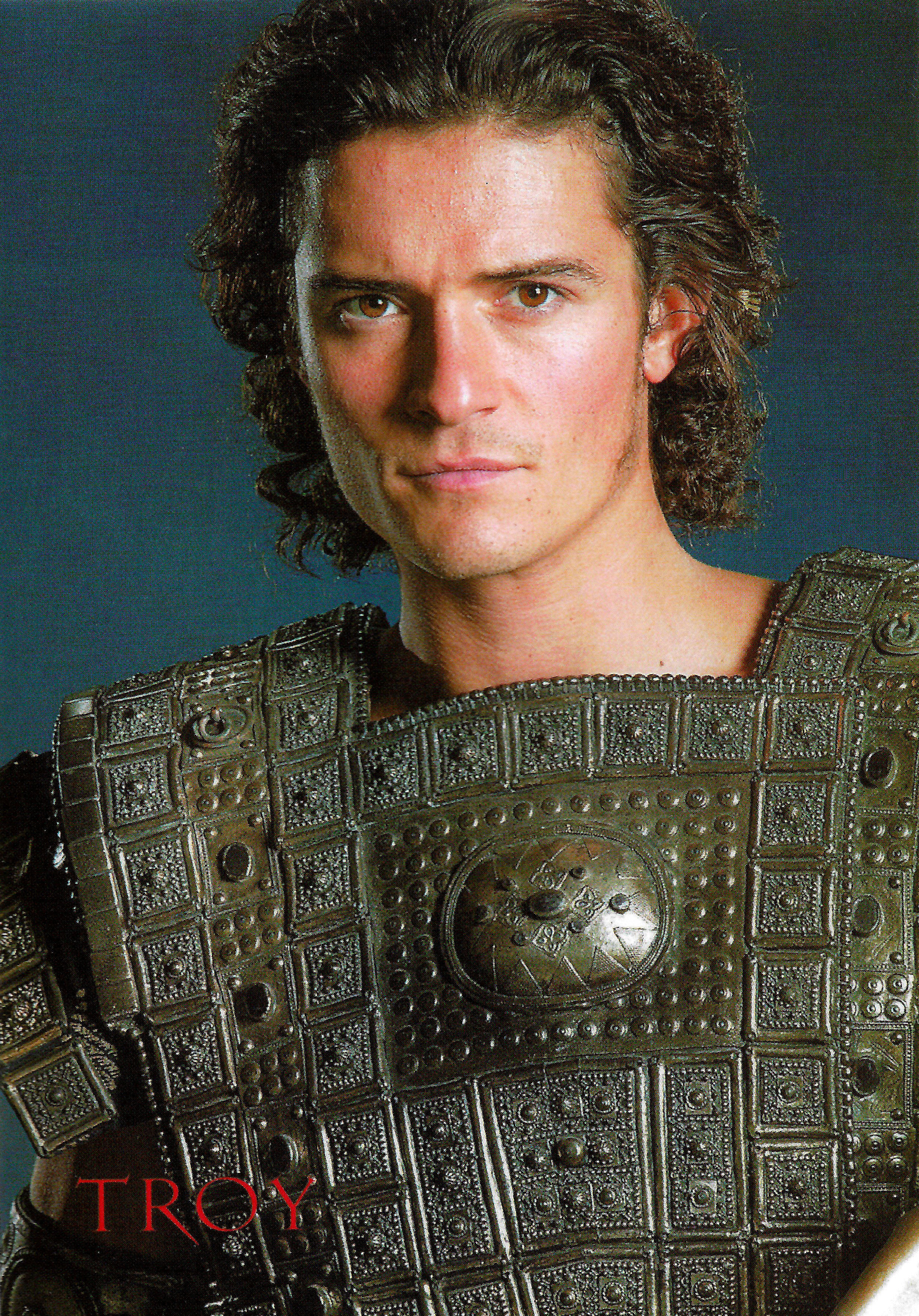This photograph features a young Orlando Bloom, particularly in his role from the film "Troy," as indicated by the movie title prominently displayed in the bottom left corner in red letters styled in the film's font. Bloom is depicted in detailed bronze-era battle armor that covers his shoulders and chest, with a glimpse of arm armor visible as well. He has curly brown hair that reaches just above his shoulders and brown hazel eyes that look directly at the camera with a serious expression. The backdrop behind him is a grayish-blue, adding to the movie's historical ambiance. The metal armor is intricately designed, evoking the ancient period of the Trojans and Spartans, contributing to a captivating portrayal of his character.